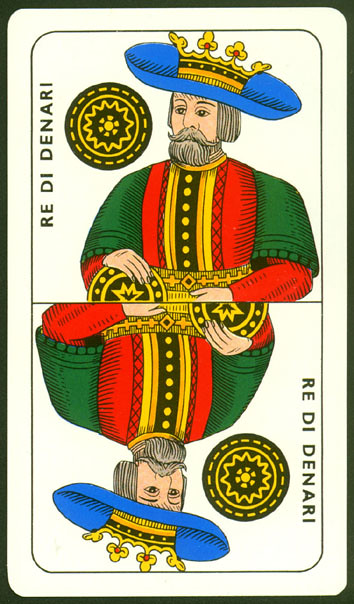This image features a detailed depiction of a playing card with a vertical rectangular shape. The card is framed by a dark green border, which is slightly thicker at the corners, followed by a white inner border and a thin green line next to it. The central section of the card is divided by a thin black line, creating two identical halves, with one half being a mirror image flipped upside-down from the other. 

The artwork within the card portrays a regal Caucasian man dressed in elaborate royal attire. He wears a blue and white hat crowned with a gold crown adorned with red jewels and detailed with black striping. His straight hair falls just below his ears, and he sports a prominent mustache and a moderately long beard.

His royal coat is richly decorated with green shoulders and a combination of red, yellow, gold, and black colors, complemented by a sash. In his hands, he holds a round, intricately designed object featuring gold and other ornate details. Additionally, another round object with black and gold decorations is positioned to the left of his head from the viewer's perspective. The inscription on the card reads "Ray R. Denari."